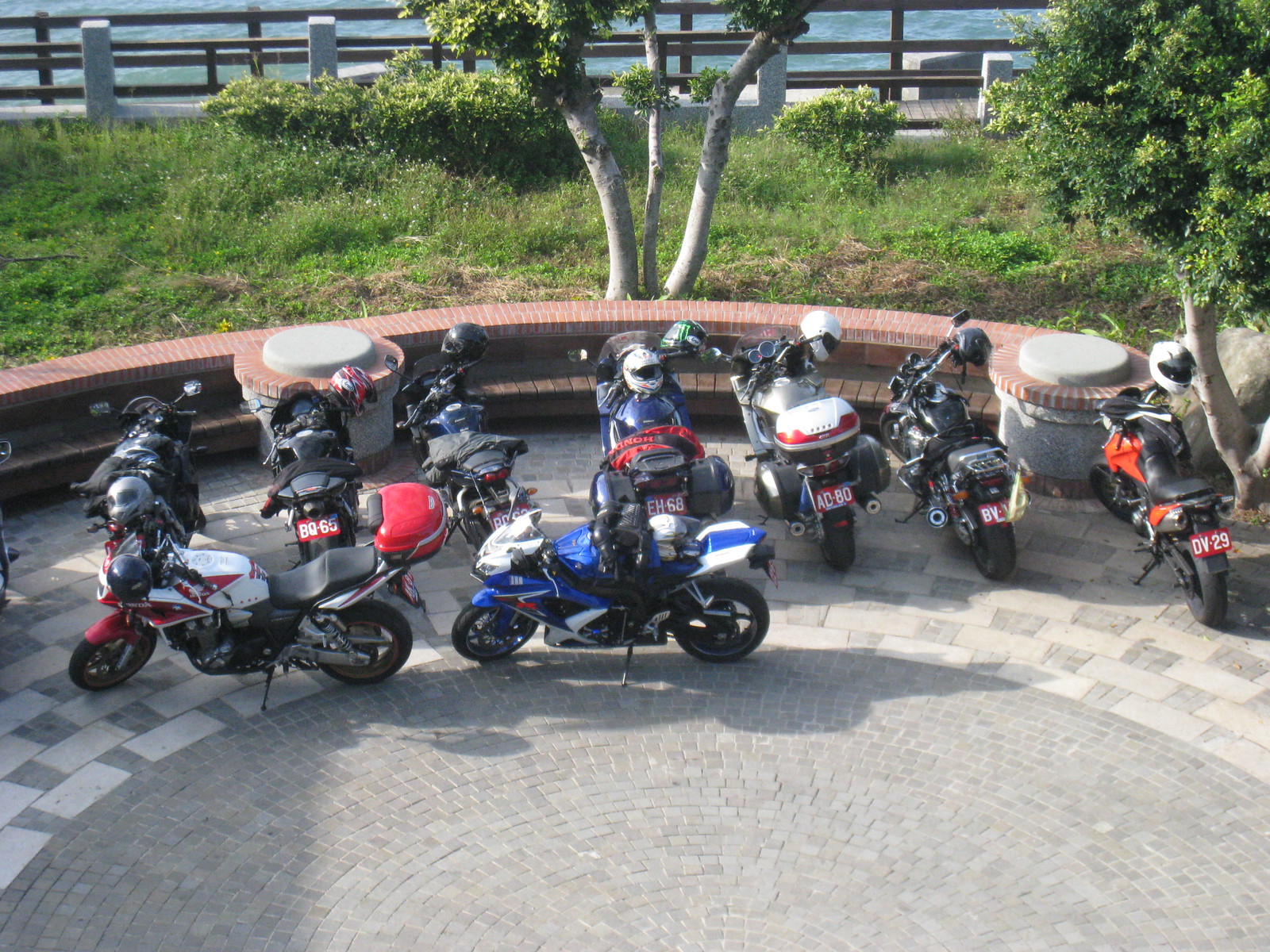This vibrant photograph captures a picturesque rest stop where nine motorcycles are meticulously parked in a circular brick-paved area. The intricate pavement design is composed of small dark gray bricks at the center, surrounded by larger rectangular cement blocks that are white with black accents. Each motorcycle is unattended, their helmets varying in color—white and black—perched on handlebars or seats, creating a uniform yet diverse spectacle. Encircling the paved area is a red brick wall that provides a structured boundary to this quaint gathering spot. Beyond this wall, lush greenery with trees, grass, and bushes adds a natural backdrop. Farther in the distance, a wooden fence leads to a walkway, where the serene blue water of what appears to be an ocean or large body of water stretches out, completing the tranquil scene. This detailed setting suggests a scenic recreational area frequented by motorcycle enthusiasts.